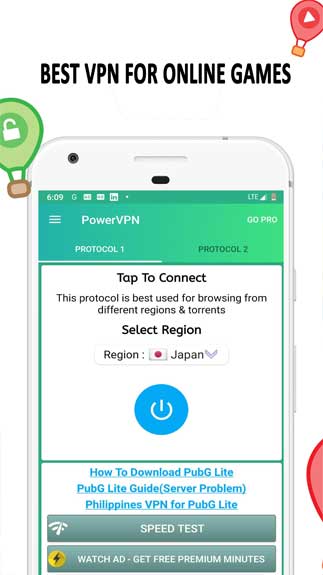The image features the following elements:

- **Top Section:** On a white background with black text, it reads, "AllCapital's Best VPN for Online Games."
  
- **Upper Right Corner:** A red hot air balloon with a red 'play' button icon is visible, with an orange basket underneath. Next to it, on the left, is a green hot air balloon displaying a white unlocked padlock icon, accompanied by a brown basket.

- **Middle Section:** Just below the balloons, a white cell phone is depicted. The phone screen is green, displaying "6:09" at the top. Icons indicate a "G-something" connectivity status and a "light" mode on the right side, along with cell bars and an almost depleted battery icon.

- **Phone Screen Display:** A green gradient bar spans from dark green on the left to light green on the right. On the left end of the bar, a menu icon with three horizontal lines is visible, alongside the text "PowerVPN." On the right end, it says "GoPro."

- **Phone Interface:** Below the bar are two protocol options: "Protocol One" (selected, in white text with an underline) and "Protocol Two" (inactive, in green text on a green background). 

- **Bottom Section:** The text on a white background instructs, "Tap to connect. This protocol is best used for browsing from different regions and torrents."

This description gives a comprehensive overview of what the image depicts.